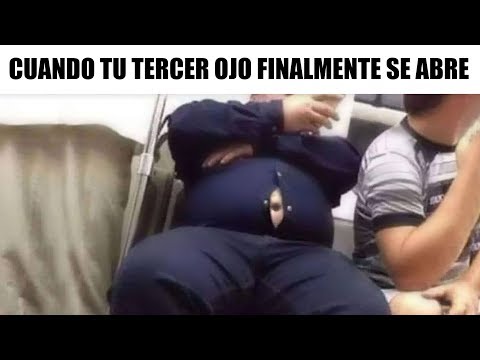The image depicts two individuals seated on what appears to be a subway train, bracketed by horizontal black borders on the top and bottom. Above the image is a caption in Spanish, "Cuando tu tercer ojo finalmente se abre," translating to "When your third eye finally opens." The main focus is a very large man dressed in a dark blue shirt and pants. His shirt is notably tight, with two open buttons around his waist exposing his navel, evidently highlighting his size. He is holding a cell phone close to his face, obscuring it from view. To his left sits a younger boy dressed in a gray, black, and white t-shirt and shorts, with his right hand also raised to his face as if he is eating. The photograph’s humor or theme might be centered around overeating or body image. The layout places the photo between two horizontal black bars, framing the scene within the context of the humorous or thought-provoking Spanish caption.